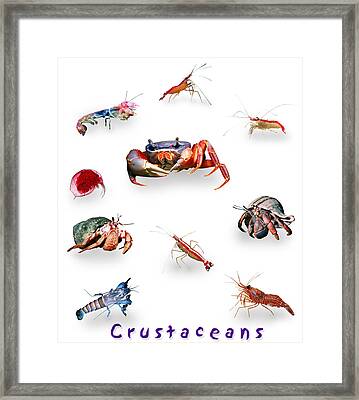This detailed artwork, encased in a light gray, inch-thick wooden frame with a rectangular shape and a white-bordered background, showcases a central prominent blue-headed crab with imposing front claws. Flanking this "big boss man" crab, there are two hermit crabs—one with a green shell and the other with a gray shell accented with a brown line. To the left of the central crab lies a small, red-smeared crustacean, and above it, a colorful rainbow shrimp. The image also features three unidentified crustaceans situated beneath these main figures. Above these, at the top of the image, are three shrimp-like creatures. At the very bottom of the picture, the word "crustaceans" is inscribed in a playful purple font, completing the lively composition of these ten diverse sea creatures.